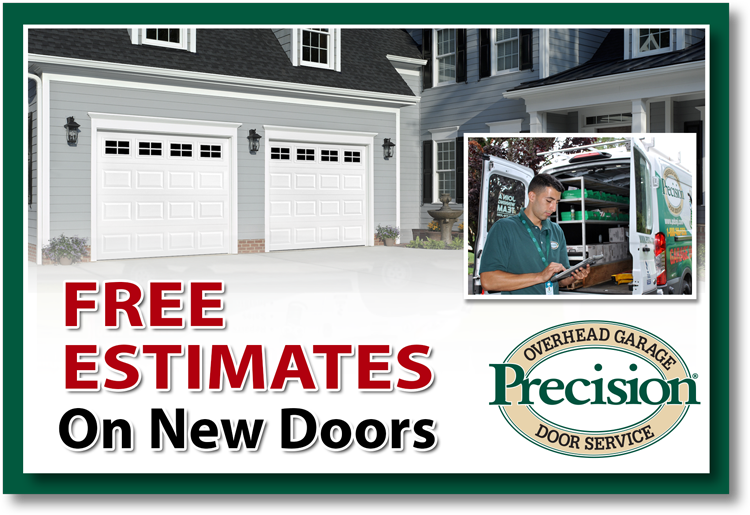The image serves as an advertisement for "Precision Overhead Garage Door Service." In the bottom right corner, there is a logo with the word "Precision" prominently displayed in green. Surrounding the logo is a beige circular background. At the top of the image, the text reads "Overhead Garage," and at the bottom, it says "Door Service." To the right, "FREE ESTIMATES" is written in bold, red capital letters, followed by "on new doors" in black beneath it.

The background features a large, multi-story gray house, potentially two houses side-by-side, each with a black roof and windows. The house features a spacious driveway in gray, two garage doors, and multiple windows, some with black window panes and white trims. Adorning the exterior are black outdoor lights. Additionally, there's a fountain positioned in the front yard.

In the foreground, there is an image of a man in a green shirt working on an iPad. He's wearing a lanyard and standing next to a truck branded with the "Precision" logo. The man is either inside the back of the truck or standing just outside it, with the truck doors open, revealing various tools and equipment inside.